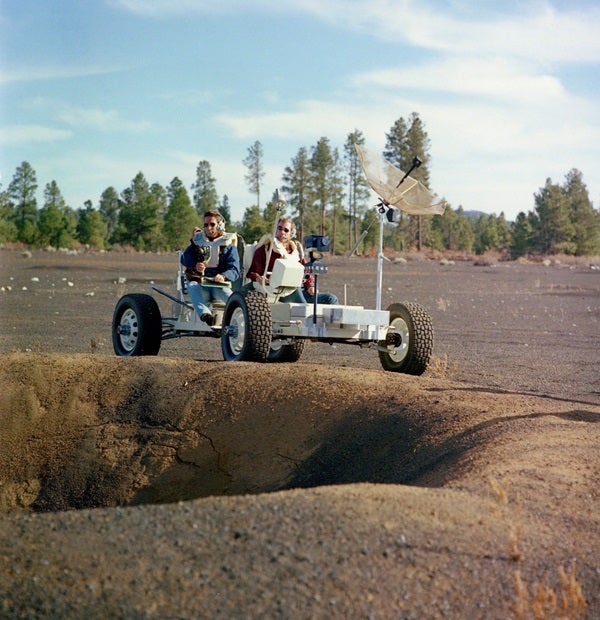In this detailed photograph, two men are seated on a white, go-kart-like structure, resembling a Mars or moon rover, equipped with four black nubby tires with white rims. The rover features an antenna-like pole mounted at the front, topped with a satellite receiver or camera. Both individuals are dressed in thick vests over their shirts; one is wearing a blue shirt and the other a red shirt. They also have headphones and microphones on their heads. In one man’s hand, there appears to be a binder or control pad.

The scene is set on what looks like a dirt area with a significant sinkhole to the left of the rover. The vehicle is positioned near this large hole in the ground. Beyond the immediate dirt area, there is a light gray-brown expanse resembling gravel, extending towards a backdrop of tall, green trees. The sky above is light blue with scattered white clouds. The overall environment suggests that the photograph was taken on Earth, as indicated by the presence of trees and the men's casual attire, not space suits.